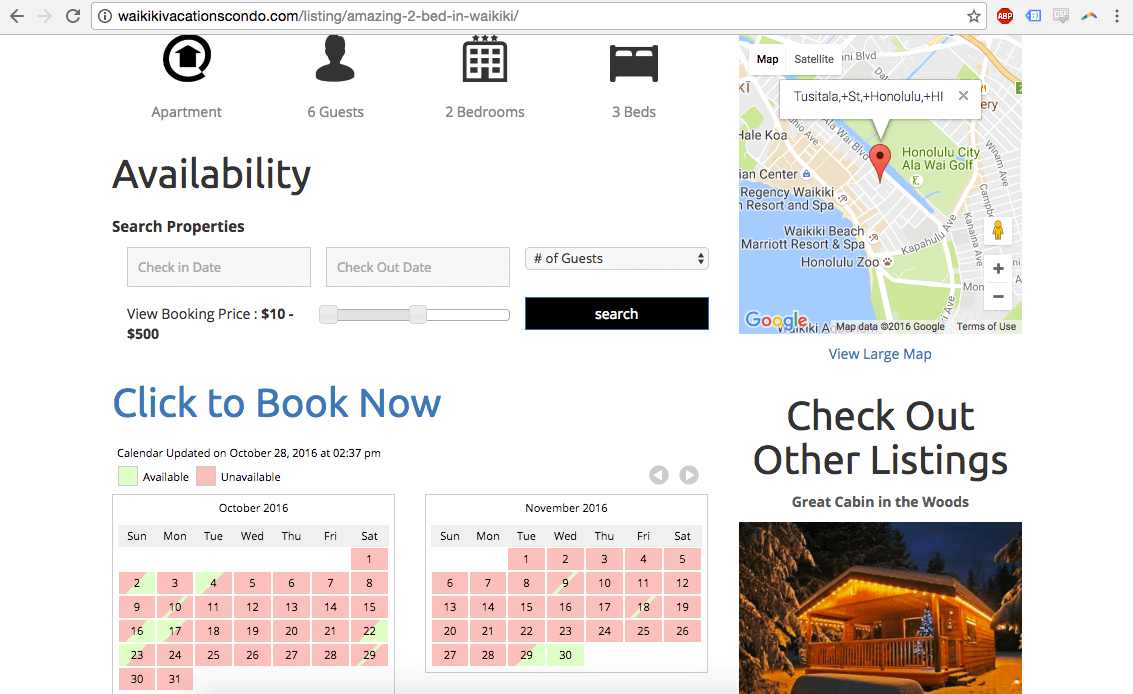**Screenshot of a Vacation Rental Website**

The screenshot captures a comprehensive view of a vacation rental webpage. In the upper left-hand corner, there's a back button, followed by a refresh button. Beside these icons is the web address: waikiki-vacations-condo.com/listing/amazing-2-bed-in-waikiki-vacations-condo.

Directly beneath the address bar, there is a website header that spans the width of the screenshot. This header includes four icons displayed side by side:
1. **Apartment Icon**
2. **Guest Icon**: indicating accommodation for up to six guests.
3. **Bedroom Icon**: specifying two bedrooms.
4. **Bed Icon**: showing a total of three beds.

Under these icons, there is a line of text labeled "Availability," followed by a smaller font phrase, "Search Properties."

Below this text are two input boxes, one labeled "Check-in Date" and the other "Check-out Date." Adjacent to these boxes is a drop-down arrow to select the number of guests.

At the bottom of the screenshot, two calendars display the months of October 2016 and November 2016, aiding in the selection of the desired dates for the stay.